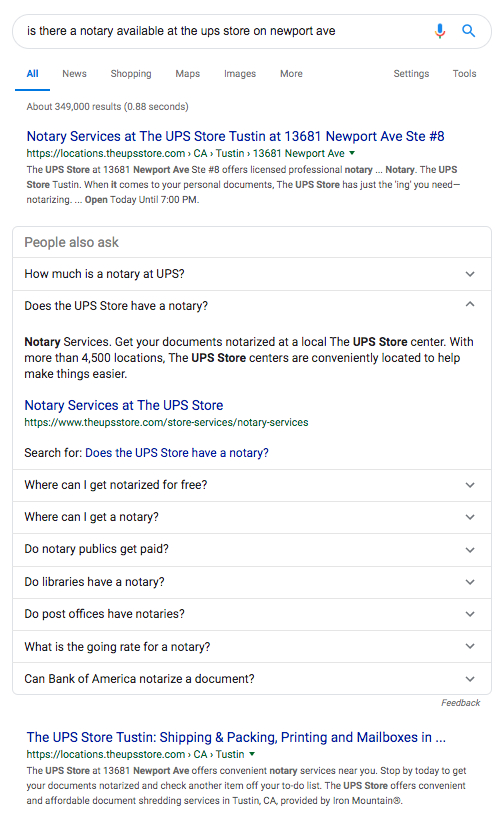This image is a screenshot taken from a tablet, depicted against a solid white background. At the top of the screen, a search bar with black text is visible. The search query reads, "Is there a notary available at the UPS store on Newport Ave?" Accompanying the search bar are the Google microphone icon and magnifying glass icon.

Below the search bar, the word "All" is highlighted in blue and underlined, with additional categories visible, including News, Shopping, Maps, Images, More, Settings, and Tools.

The first search result displayed is for notary services at the UPS Store on Tustin at 13681 Newport Ave, Suite 8. The result specifies that the UPS store offers licensed professional notary services and lists the address again as 13681 Newport Ave, Suite 8. The information continues by emphasizing the UPS Store Tustin’s reliability: "When it comes to your personal documents, the UPS store has just the thing you need: notarizing." The store's operating hours are noted, indicating it is open today until 7 p.m.

Below this result, a section titled "People also ask" appears, featuring related questions such as "How much is a notary at UPS?" and "Does a UPS store have a notary?"

This screenshot provides a clear and concise summary of the search results for notary services at the specified UPS Store location.